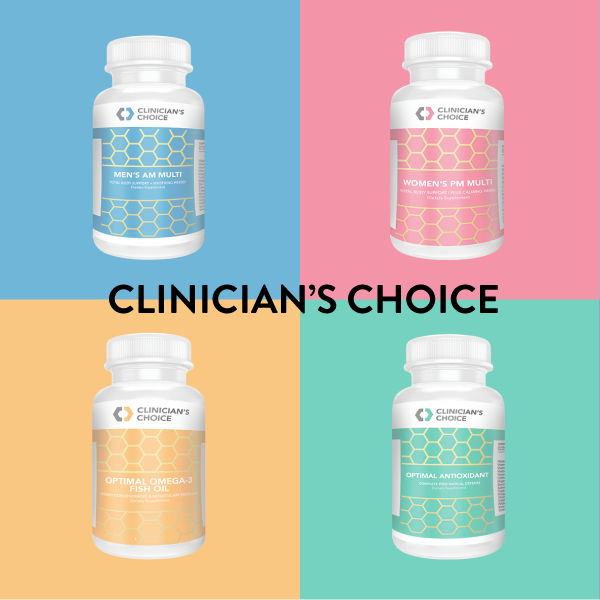The image is a photoshopped advertisement for Clinician's Choice vitamin supplements, showcasing four distinct white bottles, each positioned in one of the four differently colored quadrants of the image. The bottles are set against matching background colors: a blue background in the top left, pink in the top right, yellow in the bottom left, and green in the bottom right. Each bottle features a honeycomb design in yellow and the brand name "Clinician's Choice" at the top of the label. 

In the center of the image, the black text reads "Clinician's Choice," emphasizing the brand. The bottles are detailed as follows:
- The top left blue-labeled bottle reads "Men's AM Multi."
- The top right pink-labeled bottle reads "Women's PM Multi."
- The bottom left yellow-labeled bottle reads "Optimal Omega-3 Fish Oil."
- The bottom right green-labeled bottle reads "Optimal Antioxidants."

This visually vibrant advertisement effectively highlights the variety and branding of the health supplements offered by Clinician's Choice.